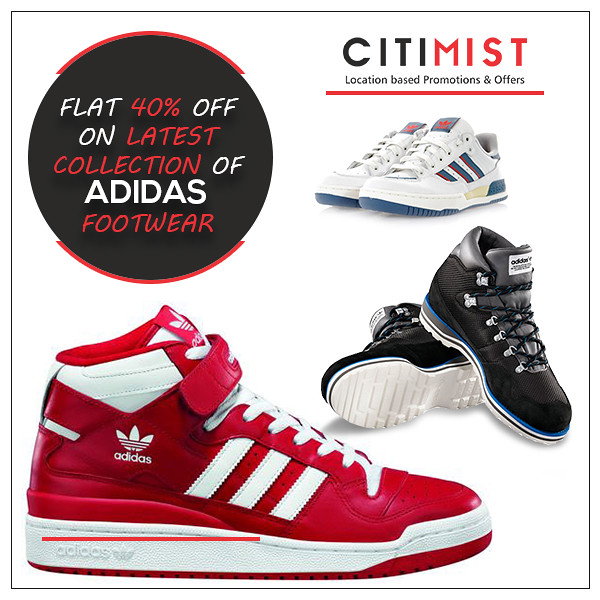This advertisement, set against a crisp white background, showcases three pairs of Adidas high-top sneakers in a visually appealing and high-resolution image. At the top left of the image is a prominent black circle containing a promotional message in red and white text: "Flat 40% off on latest collection of Adidas sportswear." In the upper right-hand corner, "City Mist" is boldly displayed, with "City" in black and "Mist" in red, followed by a subtext that reads "Location-based promotions and offers" with "offers" underlined in red.

The sneakers are arranged vertically in the central part of the image. The top pair is a sleek all-white Adidas sneaker with subtle blue and red stripes near the top. Below it, on the left side, is a stylish black and blue high-top sneaker with a distinctive white sole. The bottom left corner features an eye-catching red and white Adidas high-top sneaker. The layout and color scheme emphasize the brand's identity and the exclusive 40% discount offer, making it a compelling and informative ad for potential buyers.